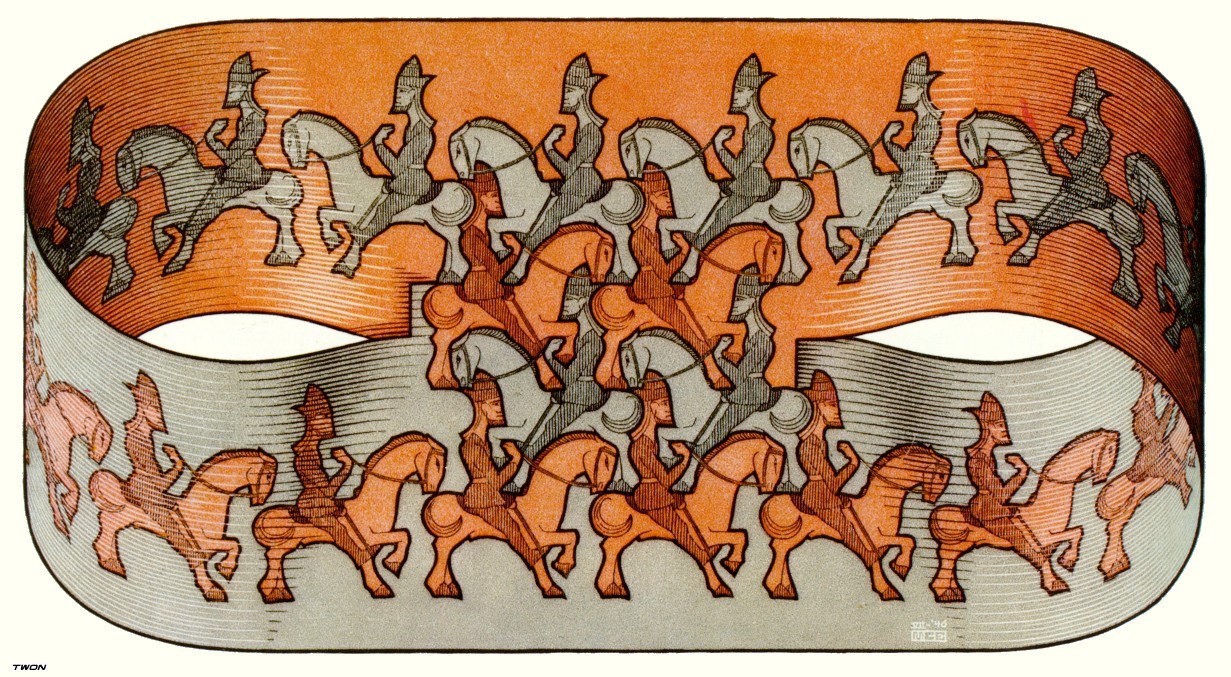The artwork depicts a detailed, rounded rectangular wrist strap adorned with an intricate pattern of horsemen in a two-dimensional style. The decoration features about 20 warriors, each wearing headdresses or helmets, and holding the reins of their horses. The image showcases two bands of these horsemen: the top band has knights in gray on horseback, moving from right to left against an orange background, while the bottom band displays knights in brown on horseback, moving from left to right against a gray background. The horses are depicted in a slight walking pose, with their right hooves raised. The entire design creates a criss-cross effect in the middle, where the pattern meets. Though there is a faint watermark with the lettering "7WGN," it is not part of the image itself.